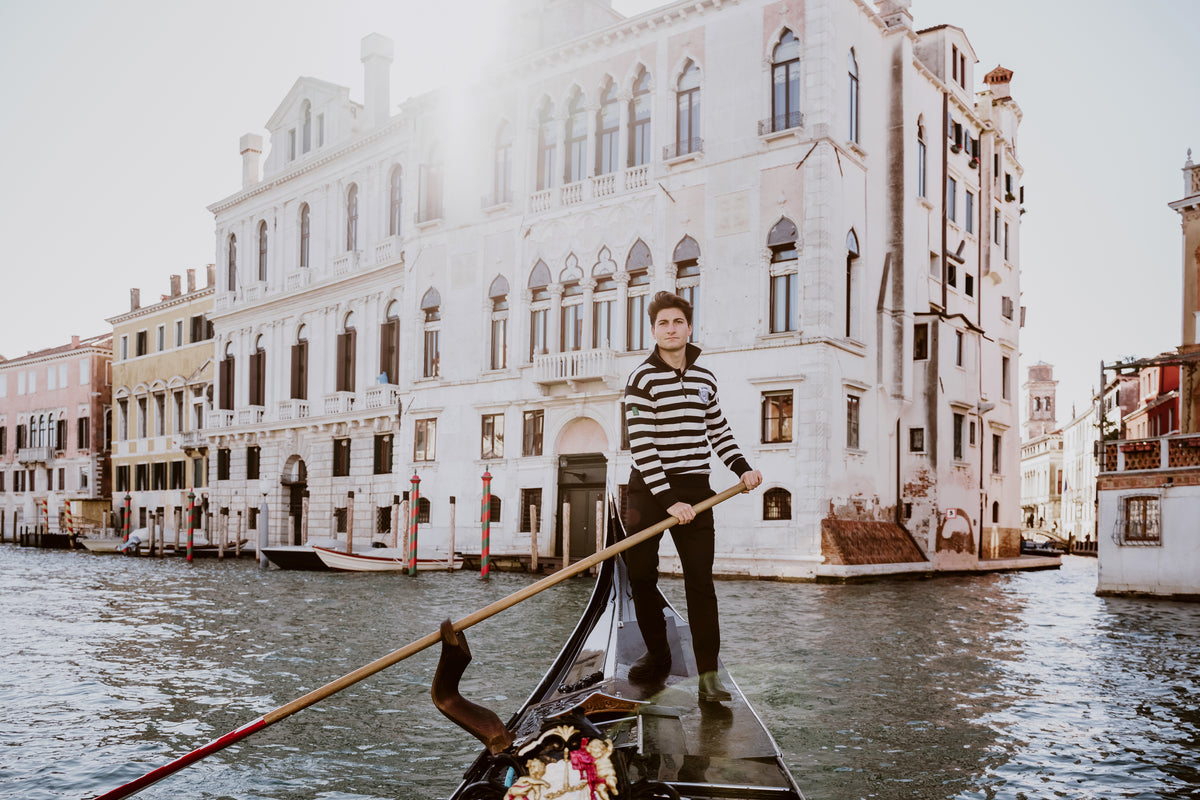This photograph captures a quintessential Venetian scene featuring a gondola navigating through the dark green waters of a canal in Venice. In the lower part of the image, the back of the gondola is visible, where the gondolier stands. He is dressed in black pants and a white and black horizontally striped shirt, which includes a partial zip from the chest upward. The gondolier, who has short brown hair, grips a long, thin paddle with a light brown wooden handle, extending it into the water on the left side of the image. He gazes toward the photographer with a neutral expression on his face.

The canal is framed by tall, three- and four-story buildings with older architectural styles. The predominant colors of these buildings are white, tan, and light pink, with intricate decorative rows of windows adding to their charm. A large, elaborate white building stands prominently in the background, flanked by a smaller white building on its right and a reddish building on its left. Additionally, a cherub-like statue is seen on the gondola, adding a touch of classic Venetian artistry to the scene.